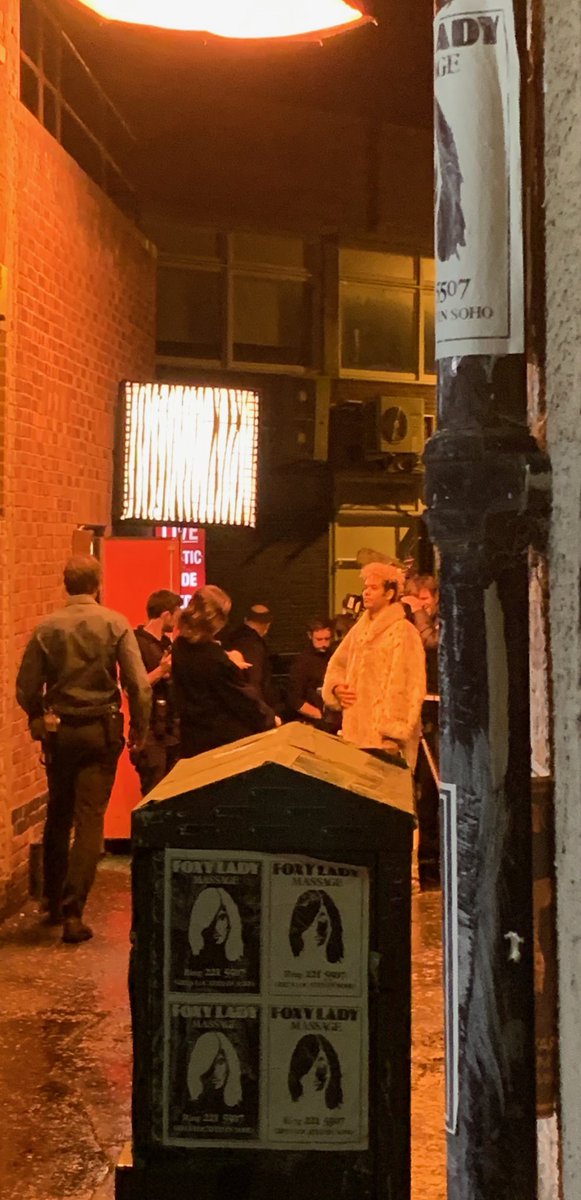The image appears to capture an immersive backstage scene or perhaps an alleyway, characterized by its narrow and confined feel. The ground is cemented, adding to the utilitarian vibe of the setting. On the right side, there's a wooden box with a paper poster affixed to it, suggesting a possible announcement or schedule relevant to the activities taking place. The image presents a somewhat washed-out quality with low light, contributing to a gritty, unpolished atmosphere.

In the background, several people can be seen, highlighting the human element within this space. One individual stands out, draped in what seems to be a luxurious mink coat, adding an element of contrast to the otherwise industrial surroundings. To the left, another figure — dressed in attire reminiscent of a security guard's uniform — walks away from the camera, contributing to the sense of movement and activity within the scene. The left side of the image is dominated by a brick wall, reinforcing the narrow confines of the setting. 

A large, bright light fixture is situated towards the left-center of the frame, illuminating parts of the image and casting shadows that add depth and texture. On the right-center side, doors are visible, possibly leading to another area, hinting at the transitional nature of this space.